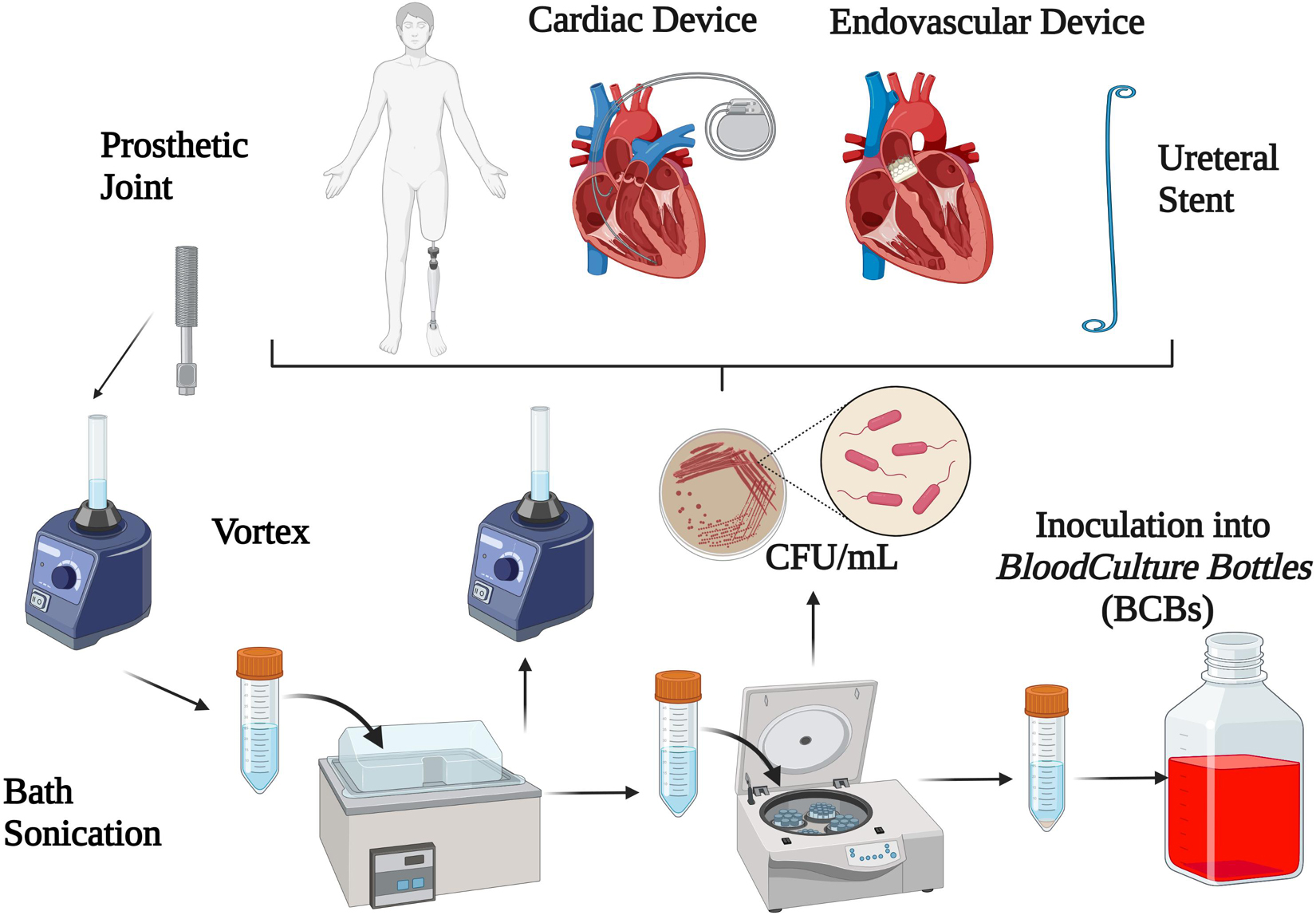The image is a detailed, hand-drawn medical flowchart against a white background, illustrating various medical devices and procedures. At the top center, there is a series of illustrations: on the left, a gray drawing of a person with a missing leg fitted with a robotic prosthetic leg; adjacent to this, two sliced human hearts are depicted in red and blue, labeled "cardiac device" on the left heart with an attached cardiac device and "endovascular device" on the right heart showing a different device inside. To the far right, there's an illustration labeled "ureteral stent."

Below these illustrations, the diagram continues with various labeled lab equipment and their processes. To the left beneath the prosthetic leg figure, there is a detailed view of a prosthetic joint, which directs attention downwards to a sequence of devices: a bath sonification machine, a vortex, and another machine that branches off into additional vials. One path from these machines leads to a series of close-ups showing bacteria, while an alternative path leads to a larger jar of blood labeled "inoculation into blood culture bottles (BCBs)." The entire flowchart methodically depicts the steps and components involved in these medical procedures.